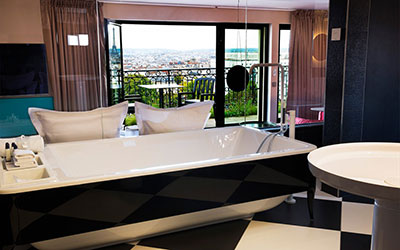This photograph showcases a luxurious, modern bathroom, featuring a striking checkered floor pattern of black and white tiles. Dominating the center of the image is a large, elegant bathtub with a white porcelain interior and a contrasting black exterior trim. To the right, there is an expansive sink, with a unique, wide, and flat design resembling a birdbath. Near the sink, a substantial faucet is present, adding to the room's sophisticated feel.

Adjacent to the bathtub, you'll find two comfortable pillows, perfectly positioned for relaxing against the tub. The right side of the photo reveals a potential sliding glass door, leading to either another tub or a shower, set against a grayish-blue wall. On the left side, a sleek flat-screen TV is visible, contributing to the bathroom's high-end ambiance.

In the background, a balcony can be seen through a glass door, furnished with a small table and chairs, offering a serene view of a sunny cityscape with smaller buildings in the distance. This area can be veiled with mauve curtains, creating an intimate and private atmosphere when desired.